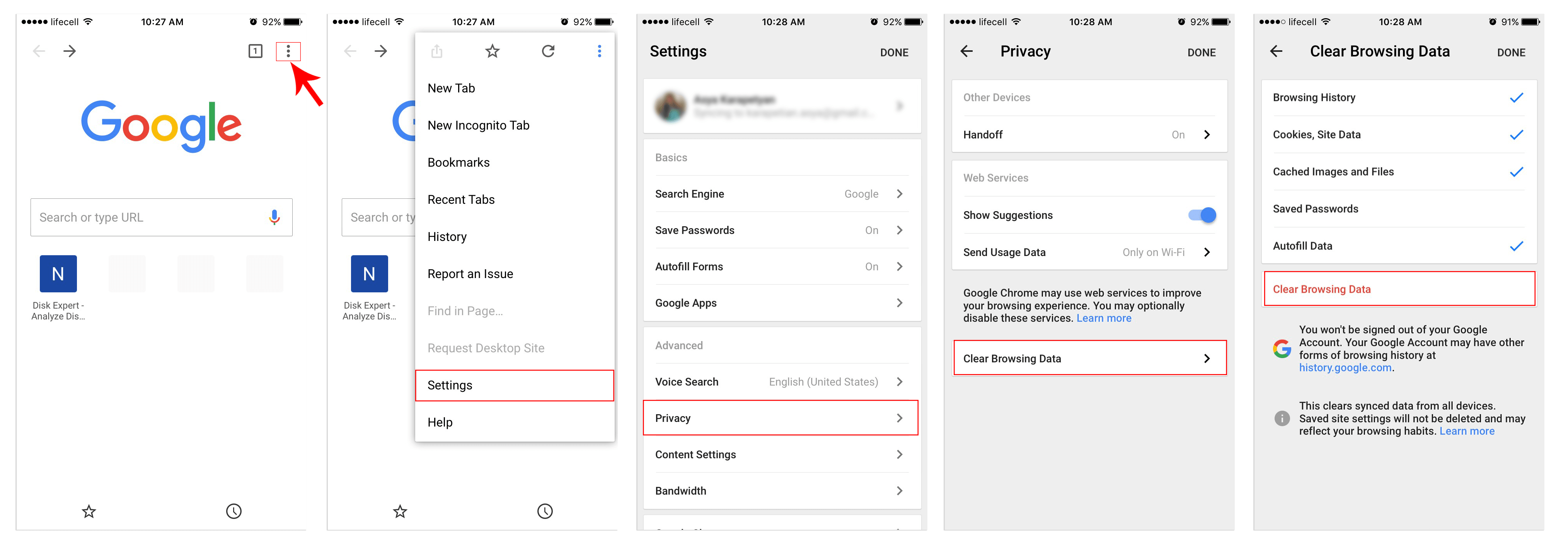The series of six screenshots provides a step-by-step guide on how to clear browsing data in Google Chrome. 

1. The first screenshot shows the Google Chrome browser interface with an arrow pointing to the three vertical dots (menu icon) in the top-right corner, indicating where to click.
2. The second screenshot displays the expanded menu after clicking the three dots, highlighted with a square around the "Settings" option, and further emphasizing it with a red circle.
3. The third screenshot shows the opened "Settings" page with another red circle specifically around the "Privacy and security" section.
4. The fourth screenshot zooms in on the "Privacy and security" section, where the "Clear browsing data" option is circled in red.
5. The fifth screenshot presents the "Clear browsing data" interface, with checkboxes for various types of data: browsing history, cookies, cached images and files, saved passwords, and autofill data.
6. The sixth screenshot concludes with instructions on clearing browsing data, underscoring the importance of ensuring all desired checkboxes are marked before clicking the "Clear data" button.

Each screenshot is accompanied by annotated instructions to guide the user through the process seamlessly.